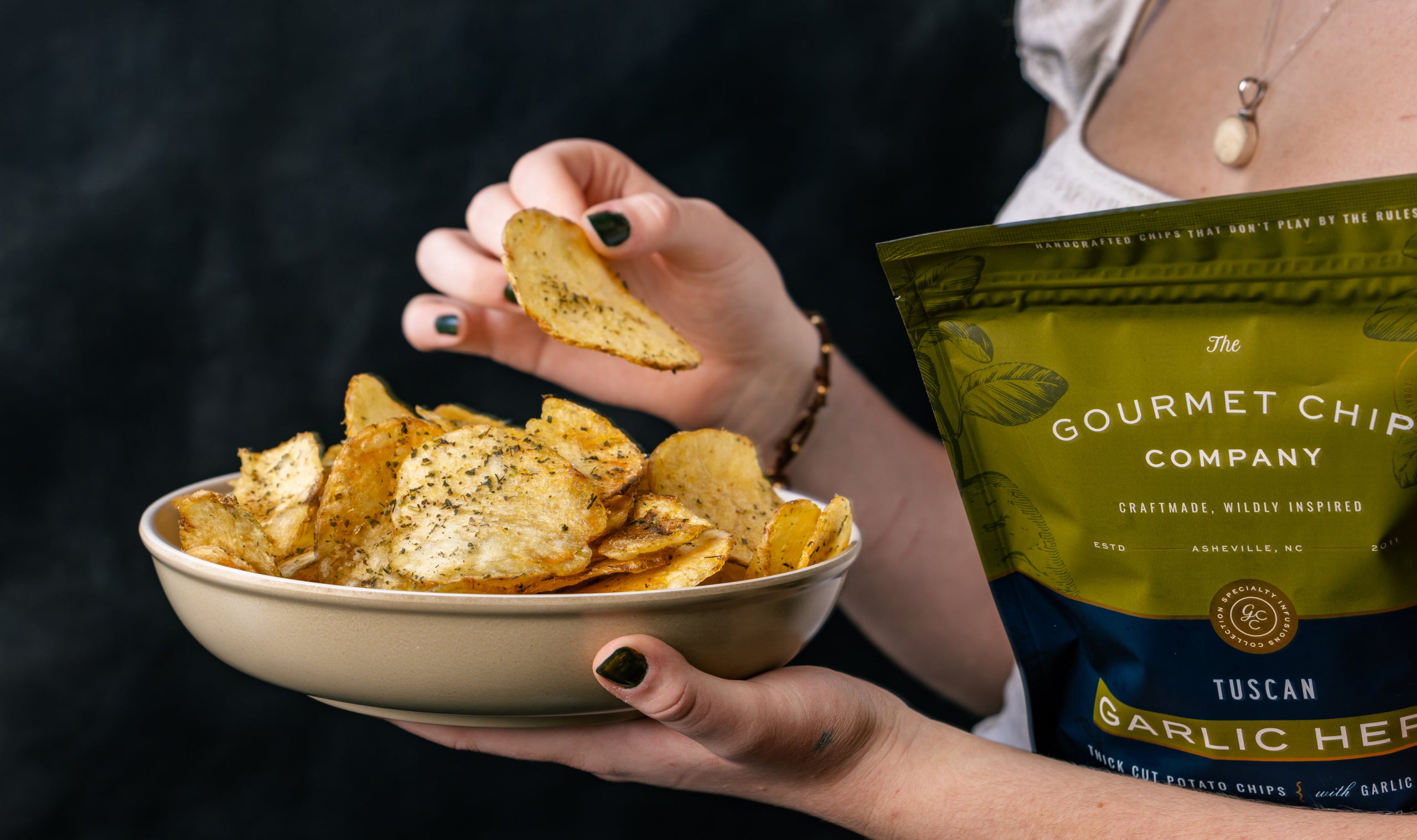A close-up image captures a pair of hands, one holding a beige bowl filled with potato chips and the other gently gripping a partially visible green and blue bag labeled "The Gourmet Chip Company - Garlic Herb." The hands, featuring fair skin and adorned with black fingernail polish and a brown and orange cloth bracelet on the left wrist, emerge from the sleeves of a white garment. The background is a stark black, making the colorful elements of the scene stand out vividly.